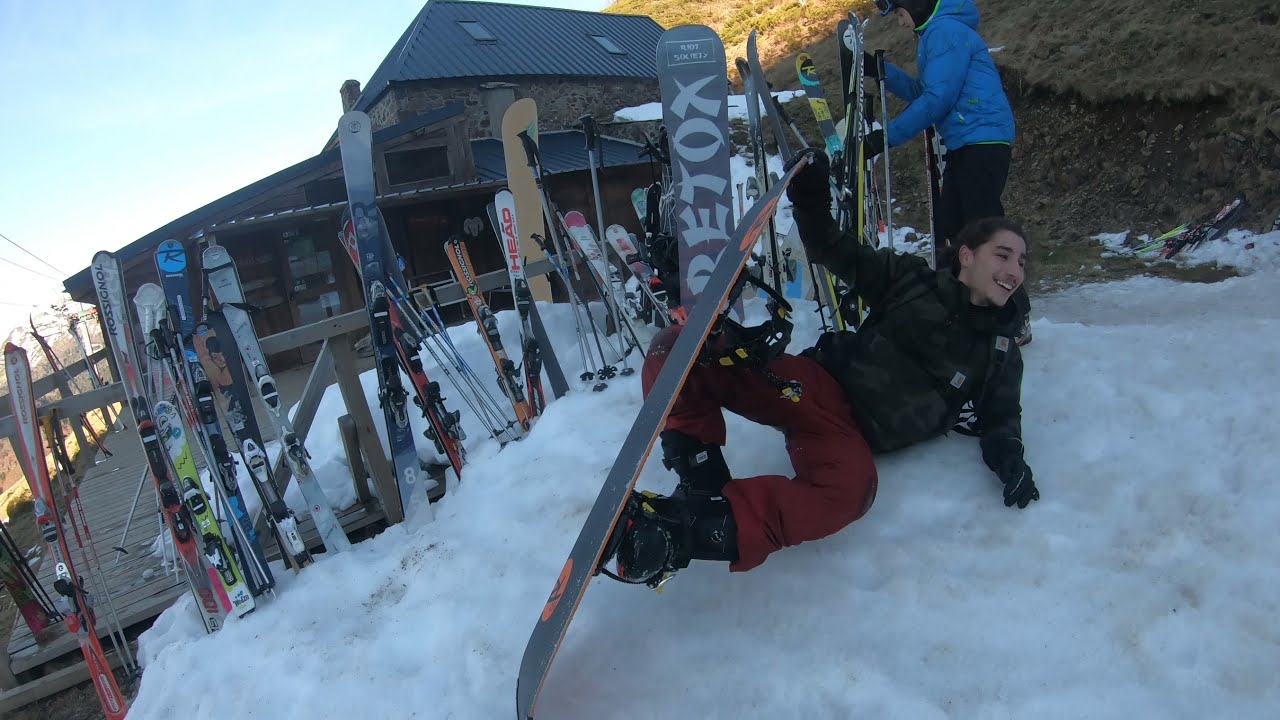The image captures a young man lying on the snow at a ski resort, posing with a snowboard. He is wearing a black jacket and red snow pants. Despite the sunshiny day, the lighting casts him in shadow, making details less clear. Behind him, a person in a blue jacket and black pants is either putting down or taking away skis or snowboards from a rack. The setting features a collection of snowboards propped against a wooden fence, which is part of a worn wooden deck connected to a stone building, likely a resort cabin. There is packed snow on the ground around the young man and the other person, with a patchy, snow-free ground in the background and green trees completing the scene. The sky is light blue, adding to the bright atmosphere of the day.